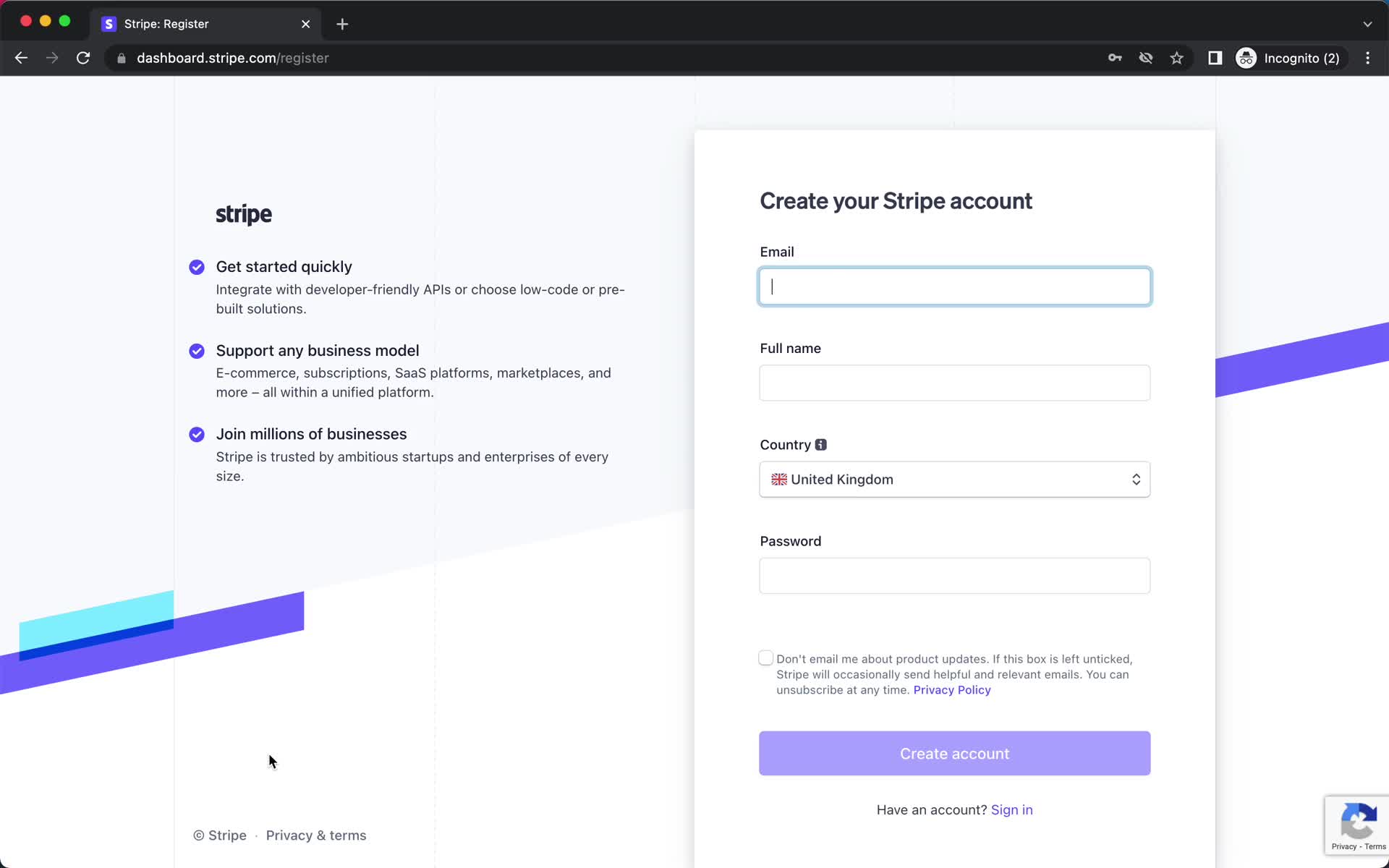The image depicts a webpage with a sleek, minimalistic design. The top section of the webpage has a black header featuring three small, horizontal dots on the left. These dots are color-coded from left to right in red, yellow, and green. Adjacent to these dots is an icon resembling a microphone, followed by a search bar. Moving to the right side of the header, there's a segment that indicates "Incognito 7" alongside an incognito mode icon and several other small icons.

Below the header, the main body of the webpage has a white background. On the left side, there is prominent branding for Stripe, marked by the following key informational points, each preceded by purple circles with white check marks:
- "Get started quickly"
- "Support any business model"
- "Join millions of businesses"

Further down, there is a visually striking element consisting of a diagonal blue line overlapping a larger diagonal purple line.

On the bottom right-middle section of the image, there's a segment dedicated to user account creation. This section includes:
- The Stripe logo
- Links for "Privacy" and "Terms"
- A prompt: "Create your Stripe account"
- Input fields for "Email", "Full Name", and "Country" (with United Kingdom selected by default)
- A password input field
- An option that reads: "Don't email me about product updates," with additional information stating that if the box is left unchecked, Stripe will send notifications and email updates

At the very bottom of this section, a prominent purple banner with white text invites users to "Create account." Below this banner, there's a reminder for existing users: "Have an account? Sign in."